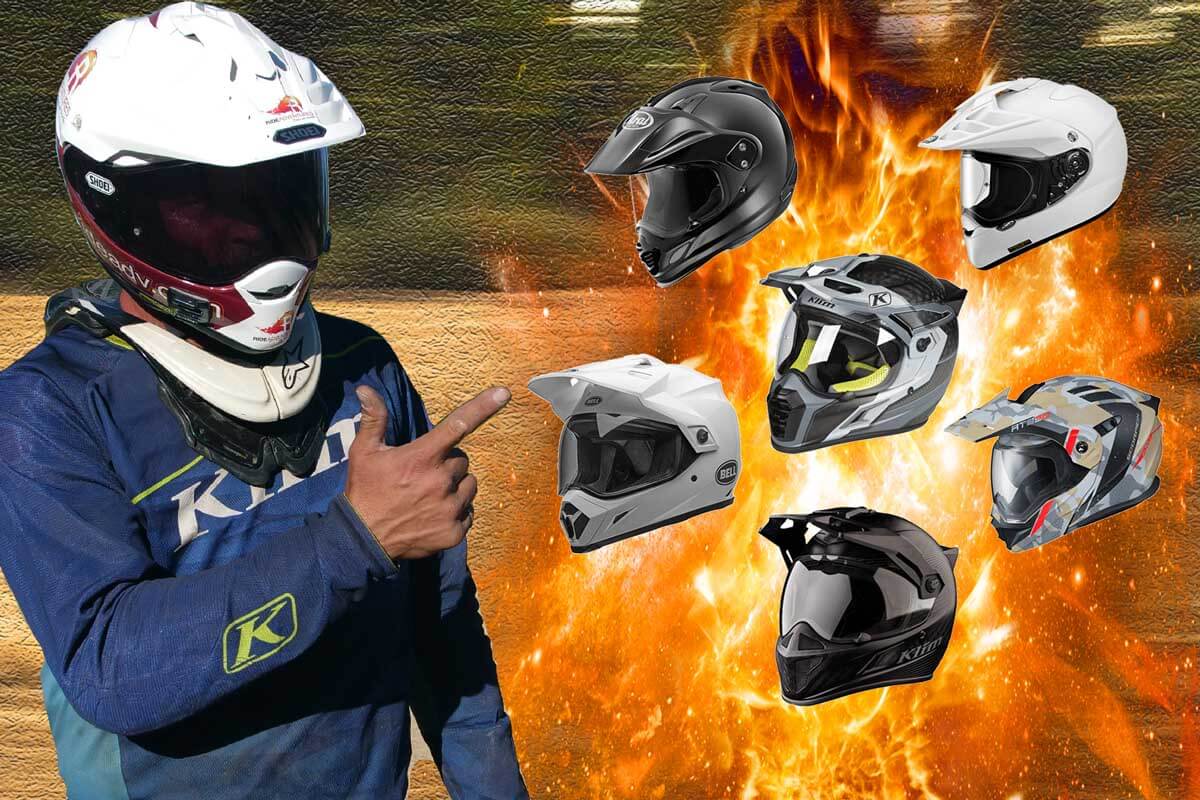In the image, a man stands on the left, wearing a long-sleeved blue jacket adorned with a yellow letter "K" on the right arm. He is pointing to the right with a dirt-smudged hand, finger extended and thumb up. His face is obscured by a white motorcycle helmet with a dark, reflective visor. To the right, six helmets float in front of a roaring, digitally-added fire, which emits orange and yellow flames dotted with small fireballs. The helmets are arranged in a vertical sequence: at the top is a black helmet, followed by a white one, a gray and silver one, another white helmet, a multicolored helmet of gray, red, and light brown, and finally at the bottom, an all-black helmet. All helmets have plastic shields and are facing left, with the fire blazing dramatically behind them.